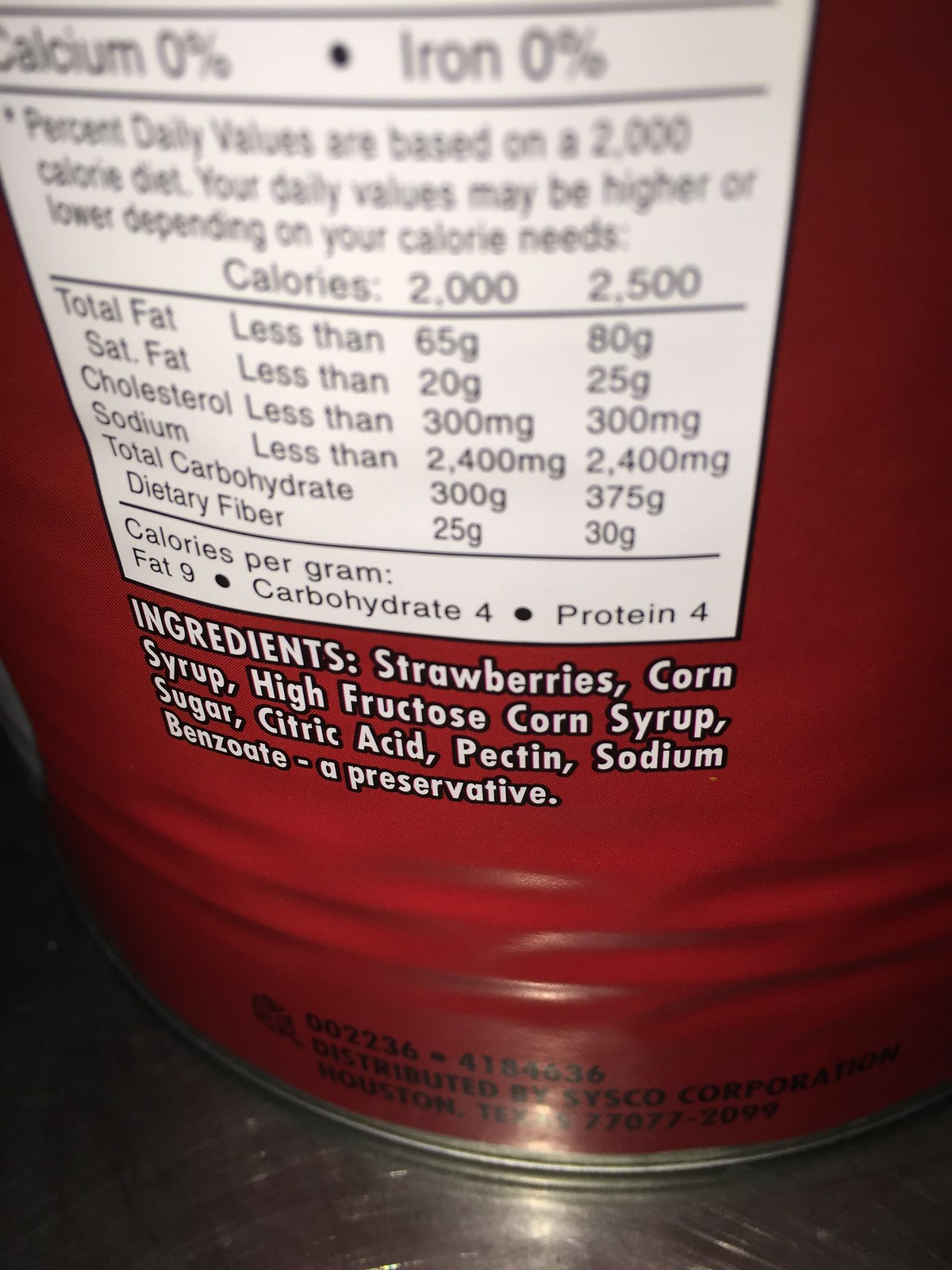This image captures a close-up of the back label of a maroon can, highlighting its nutritional facts and ingredients list. The can, which features black and white text, is set against a dark gray surface that resembles leather or metal. The clearly visible list of ingredients includes strawberries, corn syrup, high fructose corn syrup, sugar, citric acid, pectin, and sodium benzoate as a preservative. The nutritional facts indicate that the product contains 0% calcium and 0% iron. The label details additional nutritional information, such as daily values based on a 2,000-calorie diet, with specific measures for total fat, saturated fat, cholesterol, sodium, total carbohydrates, dietary fiber, and calories per gram for fat, carbohydrate, and protein. This product is distributed by Cisco Corporation in Texas.